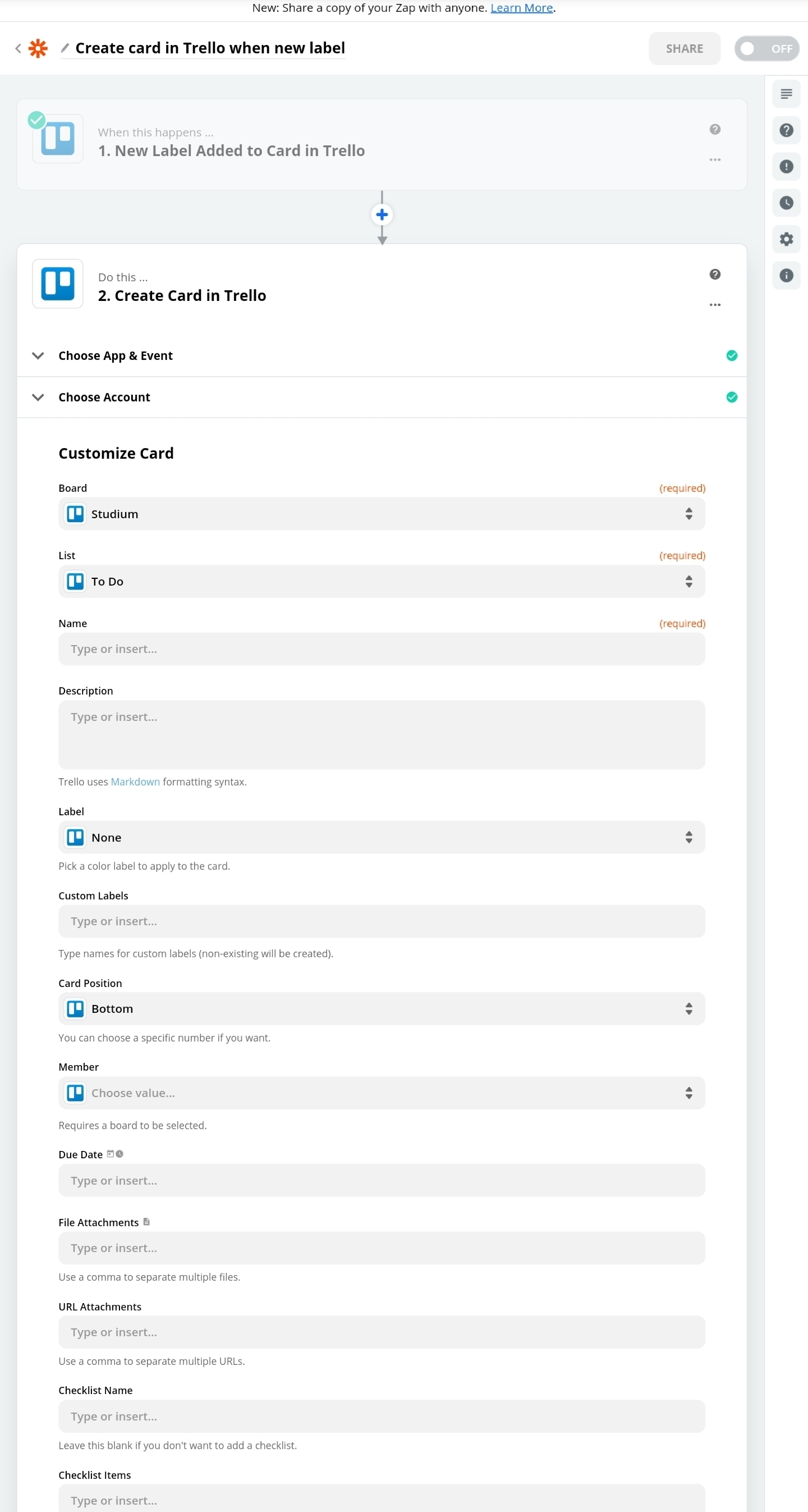**Detailed Caption for the Screenshot:**

The image is a screenshot of a text-heavy user interface within a workflow automation platform. At the top of the screenshot, there is a section titled "New: Share a copy of your Zap with anyone. Learn more." Directly beneath this, a red gear icon is accompanied by the text "Create card in Trello when new label." Below this, a circular icon with a check mark and an image resembling a page is labeled "When this happens: 1. New label added to card in Trello."

An arrow pointing downwards connects to the next section. Along this arrow, there is a white circle containing a blue plus sign. Following the arrow, on the left side, another image resembling a page can be seen with the text "Do this: 2. Create card in Trello."

Further down, a section titled "Choose app and event" is present, followed by "Choose account." The next line contains larger text that reads "Customize card." The word "Board" appears with a label indicating it is "Required." Next to it is an image of a page and the text "studium," clarified as not being "stadium." Below this, the text "List" appears, accompanied by another page-like icon and the word "to do."

Subsequent elements include "Name" with a text box that contains the words "type or insert..." A header for "Description" follows, with a text box also reading "type or insert..." and a note that "Trello uses Markdown for formatting syntax." The section labeled "Label" features a selection indicating "None," with the instruction to "pick a color label to apply to the card."

Further categories listed include options for customization such as "Custom labels," "Card position" (chosen as "Bottom"), "Member," "Due date," "File attachments," "URL attachments," "Checklist name," and "Checklist items."